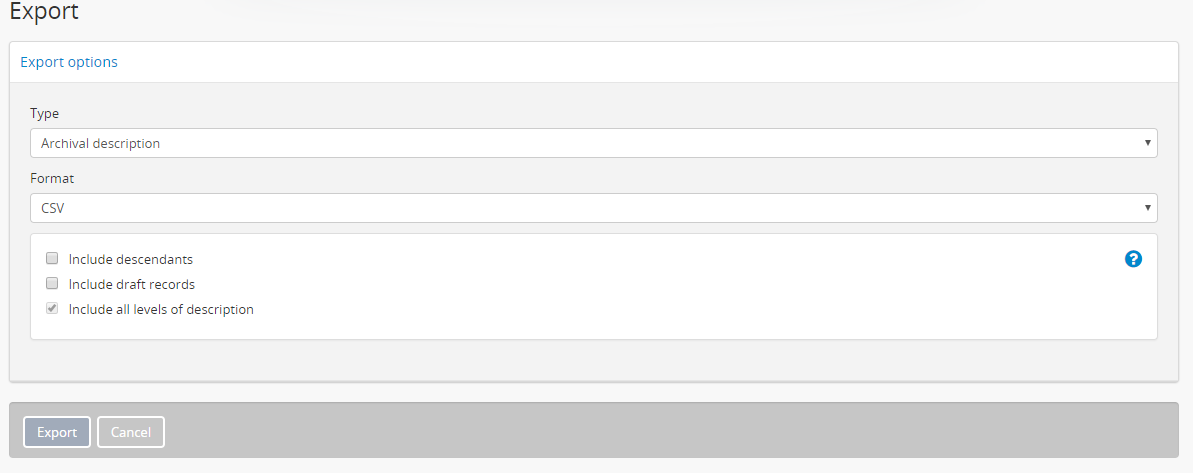The image depicts a software interface for exporting a file, presented in a long, panoramic rectangular format. Dominating the upper-left section of the image is the word "Export" in large black letters against a gray background. Below this, there is a white rectangular box containing the blue text "Export Options."

In another gray area beneath, the caption "Type" appears in black letters on the left, followed by a long, white box labeled "Archival Descriptions." This box features a downward-pointing triangle on the far right, indicating a drop-down menu.

Further down, the word "Format" is also presented in black letters, leading to an equally long white box with the acronym "CSV" in all caps inside it. This box also includes a downward-pointing triangle on the far right, suggesting another drop-down menu.

Below these fields, there is a large white box containing three gray checkboxes with corresponding options. The first checkbox, labeled "Include Descendants," is unchecked. The second checkbox, labeled "Include Draft Records," is also unchecked. The third option, "Include All Levels of Description," is checked. A blue circle with a white question mark is situated in the upper far-right corner of this section, likely serving as a help icon.

At the very bottom of the interface, there is a long gray bar. On the left side of this bar are two clickable rectangles. The first is a dark gray rectangle with white text that reads "Export," and beside it is a white-rimmed rectangular box with "Cancel" in white letters. The "Cancel" option appears grayed out, indicating it is not clickable.